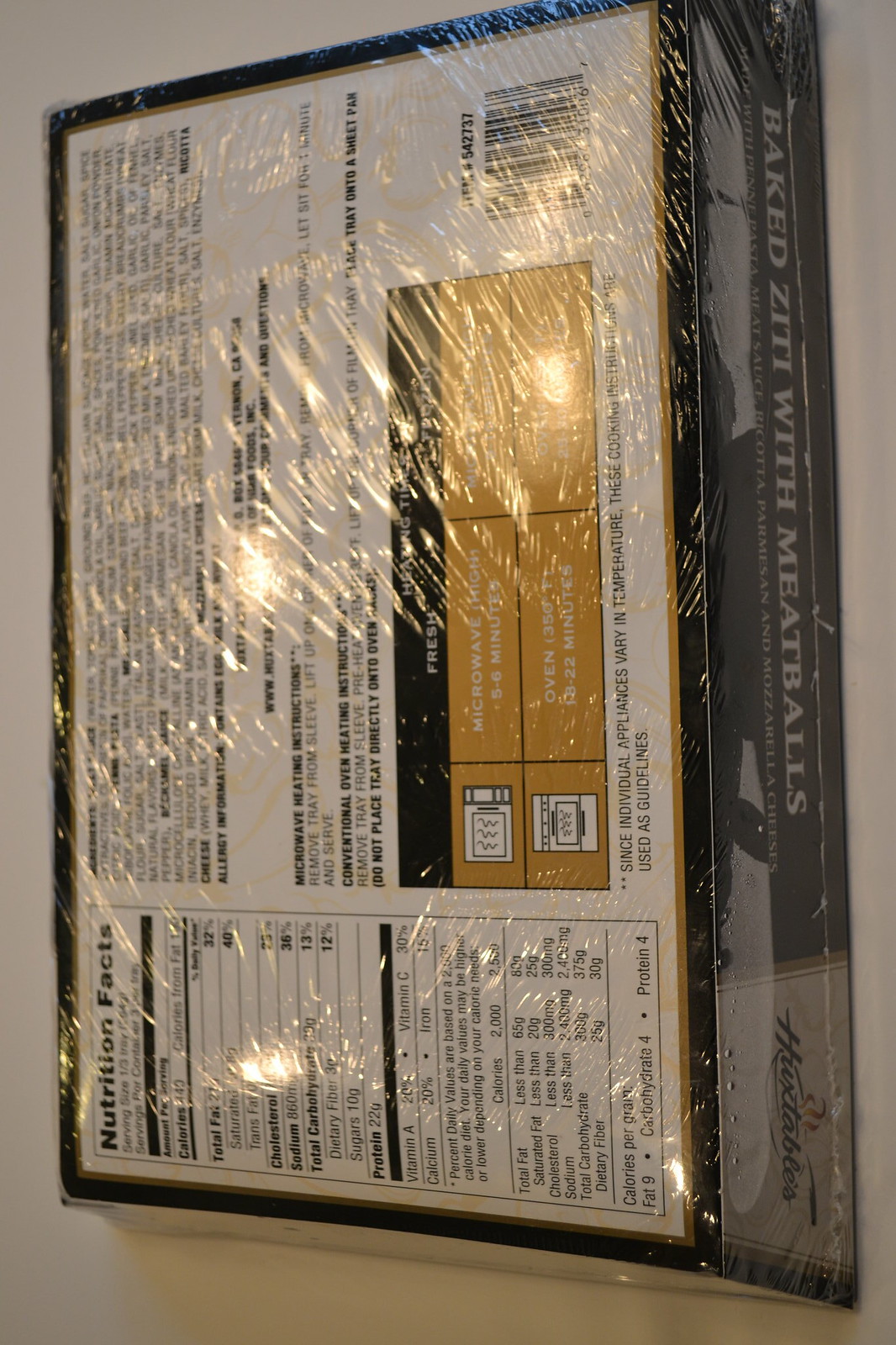This image portrays the backside of a TV dinner package, prominently displaying the details related to its contents and preparation instructions. The package itself, wrapped tightly in plastic to prevent tampering, is oriented vertically. A monochrome backdrop accentuates the shadowing and light reflections, adding to the clarity of the displayed information. The centerpiece is the label reading "Baked Ziti with Meatballs" in white text on a contrasting black background. The left section of the package features a comprehensive nutritional facts label, although the specific details are not discernible in the image. Adjacent to the nutritional information, the instructions for cooking the meal are printed in black text on a white background. These instructions include both microwave and oven options, illustrated with respective icons. The package's border is rendered in black and gold, adding a touch of elegance to the otherwise utilitarian design. The top right corner of the box is populated with multiple small text sections detailing the ingredients, echoing the practical theme evident in the rest of the package.